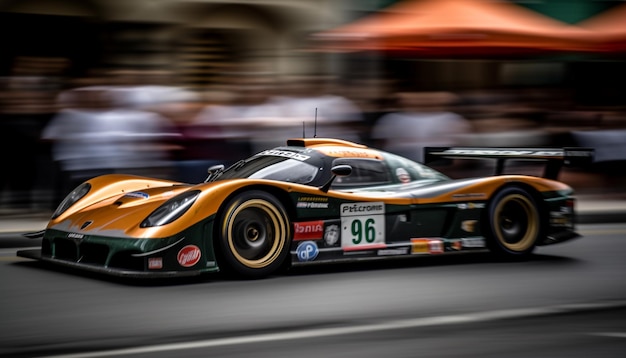The image captures a high-end race car, possibly an Indy car or a high-performance Formula car, speeding down a track. The car's aerodynamic design and significant downforce are evident, featuring a bright orange top and a dark green to almost black bottom half. The motion blur in the background, including blurred bystanders under a red tent and streaks of blurred lines, emphasizes the car's incredible speed. The car, labelled with the number 96 on its side, boasts golden-rimmed wheels and numerous sponsor stickers. It also features a prominent rear wing supported by two beams, adding to its sleek and powerful appearance. The driver sits very low, enhancing the car's streamlined build akin to a Corvette or Ferrari. The overall composition of this photograph brilliantly conveys the high velocity and dynamic motion of the race car.